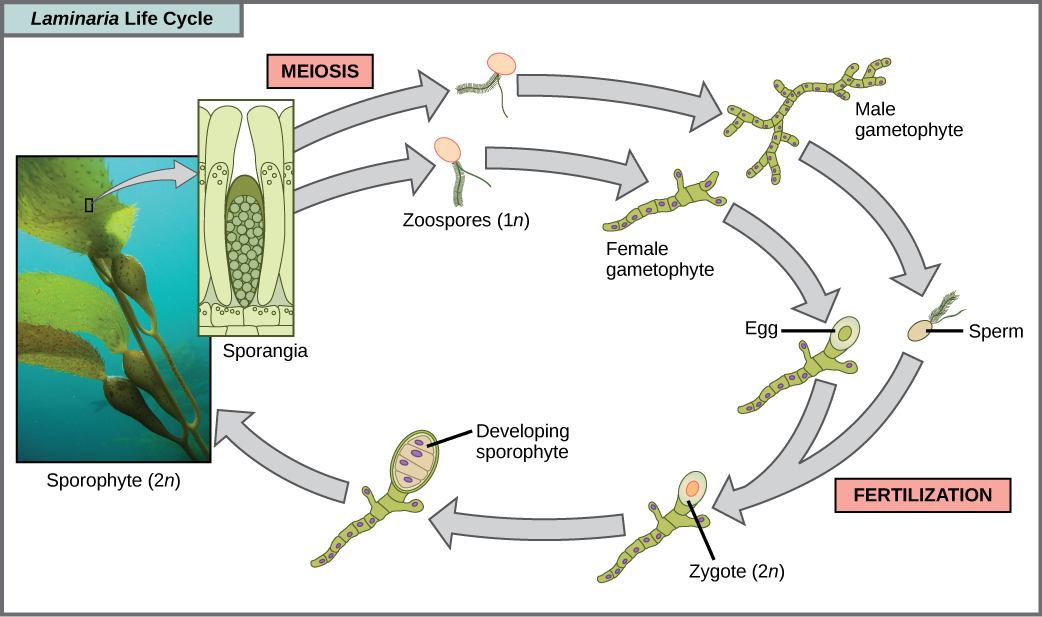This detailed diagram illustrates the Laminaria life cycle, an oceanic plant species. At the top left, a blue rectangle with black font prominently labels it as "Laminaria Life Cycle." Below this, a photograph depicts the green underwater sporophyte plant, accompanied by an arrow pointing to a detailed drawing labeled "sporangia," an internal structure of the plant. The diagram features arrows arranged in a clockwise circular pattern, highlighting various life stages. A pink rectangle labeled "meiosis" initiates the process. Subsequent stages include "female gametophyte" and "male gametophyte," followed by "sperm," "egg," "fertilization," "zygote," and "developing sporophyte." This cyclic progression ultimately returns to the initial sporophyte image, completing the life cycle. Alongside, additional stages such as "Zoo Spores" are depicted, and various descriptive boxes explain the fertilization and developmental phases with corresponding graphics.